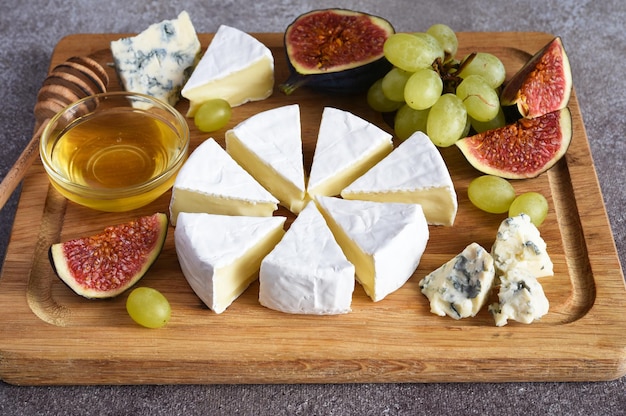This image features a beautifully arranged wooden charcuterie board, showcasing an array of cheeses, fruits, and a honey dip. The board itself is crafted from a wooden rectangular piece, possibly resembling butcher's block, and is set on a dark granite countertop. Centered on the board is a wheel of brie cheese, cut into multiple triangular pieces to reveal its creamy yellow interior and soft white exterior. Surrounding the brie are various chunks of cheese, including pieces with blue mold, likely blue cheese, and wedges of brie.

To the upper right, a small batch of green grapes on the vine is prominently displayed, with several singular grapes scattered throughout the board. Adding to the fruity selection, slices of cantaloupe and figs with a dark exterior and a pinkish interior are placed around the cheeses. Anchoring the left side of the board is a glass bowl of honey accompanied by a honey dipper, inviting guests to pair the sweet nectar with the cheeses and fruits. This meticulously arranged charcuterie board presents a harmonious blend of savory and sweet elements for a visually appealing and delightful culinary experience.